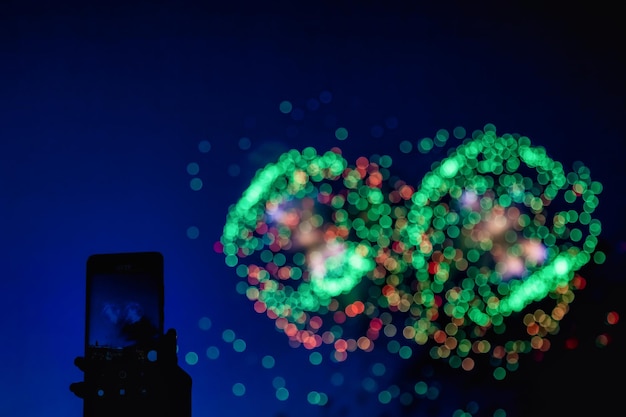In this abstract nighttime photograph, the scene is dominated by a dark, almost black and navy blue sky, giving the image a deep and mysterious backdrop. The top right portion is particularly dark, contrasting with the burst of color towards the middle and right side of the image. Here, an array of green, red, orange, and occasional yellow lights sparkle like scattered stars, with green being the most prominent. These lights appear in two distinct clusters – one towards the far right and another near the center, forming ethereal "clouds" of color. Amidst this dazzling display, likely fireworks or perhaps festive decorations, there's a dark silhouette on the bottom left: the clear outline of a hand clutching a phone, seemingly capturing the mesmerizing scene. Despite the blurriness of the photograph, this silhouette stands stark against the navy blue, adding a sense of narrative to the abstract composition.